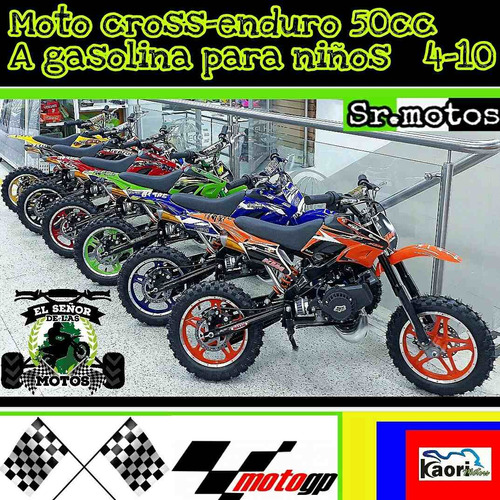The image prominently displays a row of colorful, dirt bikes arranged neatly in the center, directly in front of what appears to be a bike shop setting. The dirt bikes, or motocross bikes, are decked out in an array of vibrant colors including orange, blue, green, red, yellow, and black. At the top of the image, there is bright green text in a foreign language that reads "Motocross Enduro 50cc a Gasolina para Niños 4-10," among other phrases. Below the bikes, in the bottom left corner, there are two black and white checkered race flags crossing each other with the MotoGP logo in red and black letters. The background reveals a glass wall and a staircase, further solidifying the setting as a professional bike shop that specializes in selling motocross bikes for various age groups.